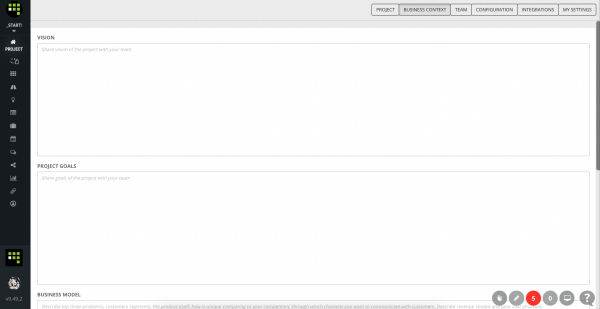This image, captured from a webpage, displays a user interface with a structured layout. On the left side of the screen, there is a vertical navigation panel enclosed in a black rectangle, making the icons within it prominent. The panel begins with a "Start" area, followed by sections labeled "Project". This vertical series consists of various icons extending downwards until reaching a space that features a distinct icon. This icon is composed of three green boxes at the top, a white box and two green boxes in the second row, followed by a single green box.

At the bottom of this black panel, a similar icon can be seen, maintaining visual consistency within the layout. Moving to the central part of the image, there's a larger rectangular text space labeled "Vision," prompting the user to "Share your vision here." Adjacent is another sizable empty rectangle designated for inputting "Project Goals" to be shared with the team. Lower on the page is another section for detailing the "Business Model."

Across the bottom of the image, there is a row of smaller icons, starting with two grey icons, followed by one red icon, and concluding with three additional grey icons. The overall design is clean and organized, guiding the user intuitively through different sections intended for input and navigation.